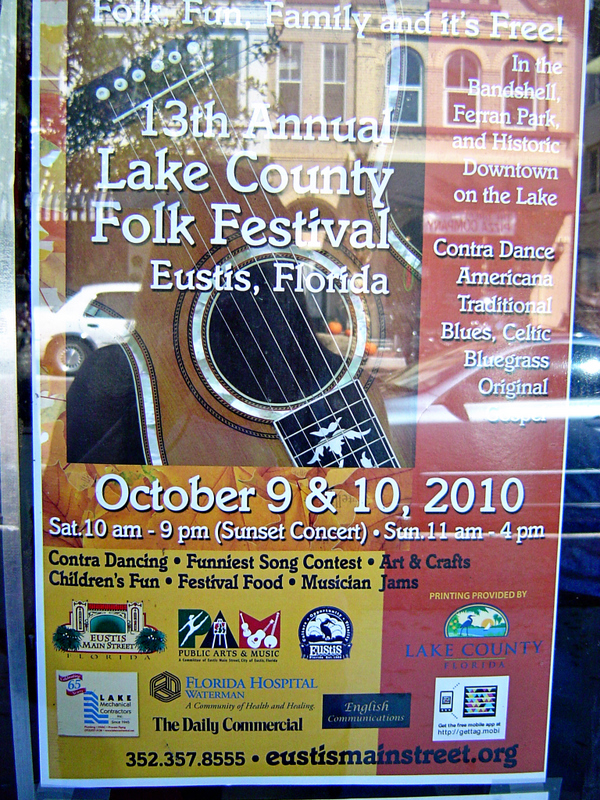This full-color photograph captures a poster for the 13th Annual Lake County Folk Festival held in Eustis, Florida through a window, with reflections revealing nearby buildings and parked cars but no people. The poster prominently announces "Folk, Fun, Family, and it's Free" at the top, with a backdrop image of a guitar. This event is set to take place in the Bandshell Park, a historic area downtown by the lake, on October 9th and 10th, 2010. Saturday's festivities run from 10 a.m. to 9 p.m., ending with a sunset concert, and Sunday's activities continue from 11 a.m. to 4 p.m. The festival promises a vibrant mix of musical genres including traditional blues, Celtic, and bluegrass, along with Americana and original compositions. Attendees can enjoy contra dancing, a funniest song contest, arts and crafts, children's activities, festival food, and musician jams. For more information, the poster lists contact details including phone numbers and a website.